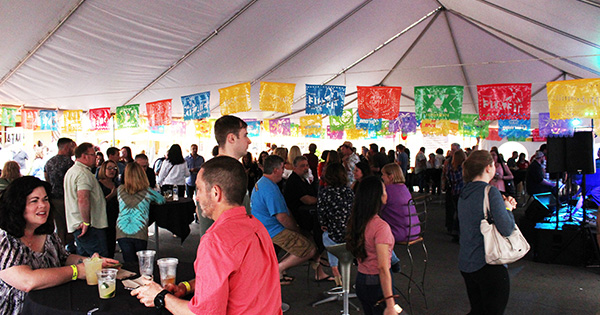This image captures an outdoor musical festival taking place under a large white tent. The tent’s ceiling, supported by a metal mesh frame with several poles, arches from left to right. Bright sunlight filters through the tent's open sides, indicating a lively daytime setting. Inside, numerous people are seated around tables adorned with drinks, engaged in conversation, and enjoying the festive atmosphere. Colorful banners in red, green, yellow, blue, and purple stretch across the tent, adding to the vibrant scene. 

In the foreground, a woman with shoulder-length black hair in a black and white dress sits on the left, facing a man with short dark hair in a pink shirt, his left arm resting on the table, and wearing a black watch. Behind him stands another person facing right. To the bottom right of the image, another woman with long black hair faces away from the camera, while beside her a woman with shorter brown hair in a gray shirt and a light-colored bag over her right shoulder also looks away.

Towards the back, more people are gathered, seated and standing, suggesting a bustling crowd. In the distance, the focus shifts to a stage lit with blue lights, equipped with sound equipment and speakers, drawing the collective attention of the festival-goers. The atmosphere is festive, communal, and vibrant, capturing the essence of a joyful outdoor musical celebration.